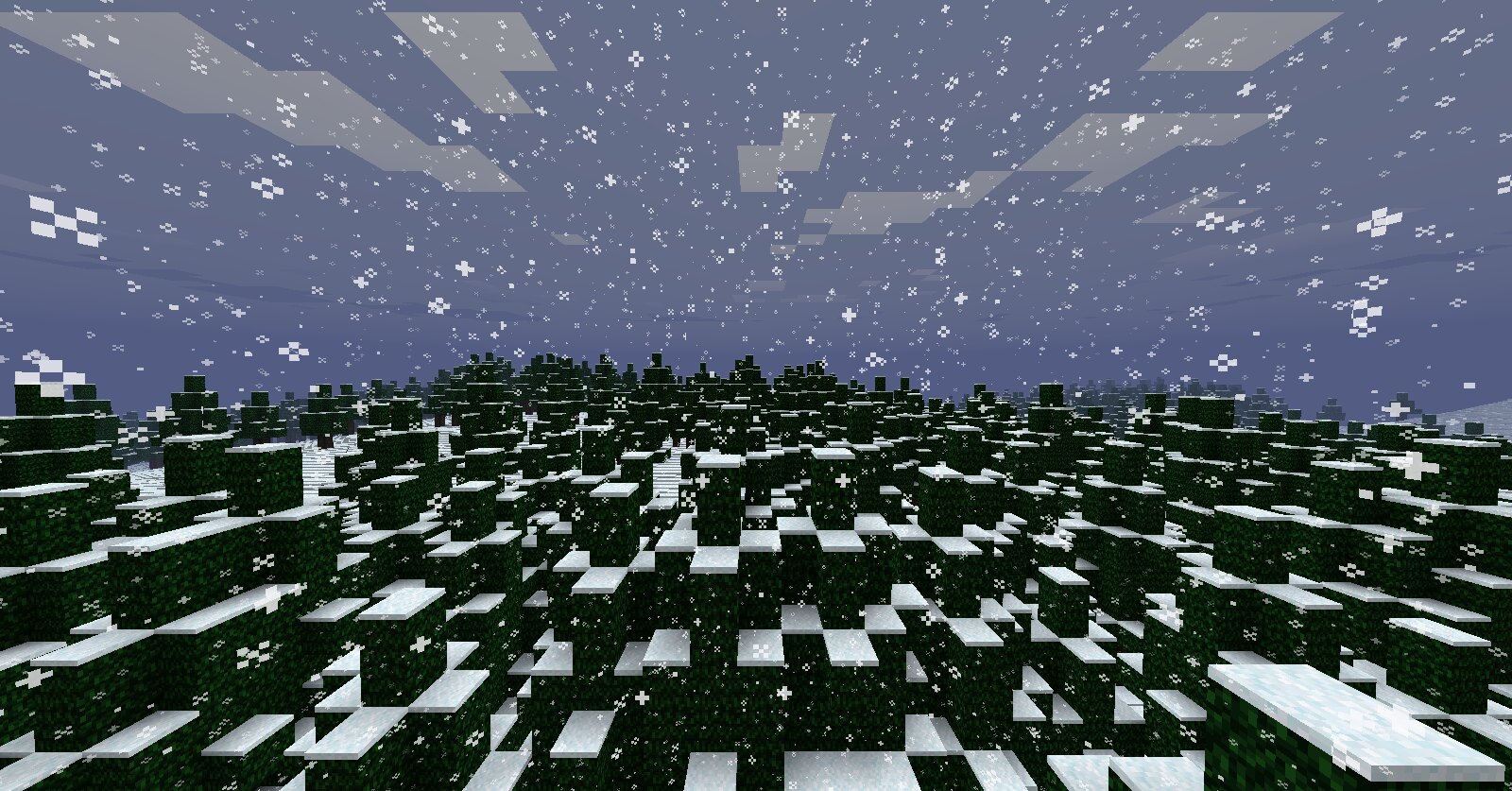The image appears to be a computer-generated scene from the popular video game Minecraft, depicting a snowy taiga biome forest. The landscape is composed of dark green tree blocks, each topped with a layer of white, mimicking freshly fallen snow. Above, the sky is a dim grey-blue, peppered with square-shaped, white pixelated clouds. Snowflakes, also pixelated, resembling tiny checkerboard squares and crosses, are falling from the sky, adding to the wintry atmosphere. The straight lines of the cubes and the overall pixelated style clearly indicate the artificial, CGI nature of the image, with reflections creating an illusion of clouds. The scene extends into the distance, filled entirely with these distinctive Minecraft blocks, illustrating a vast, continuous snow-covered forest under a serene, snowy sky.